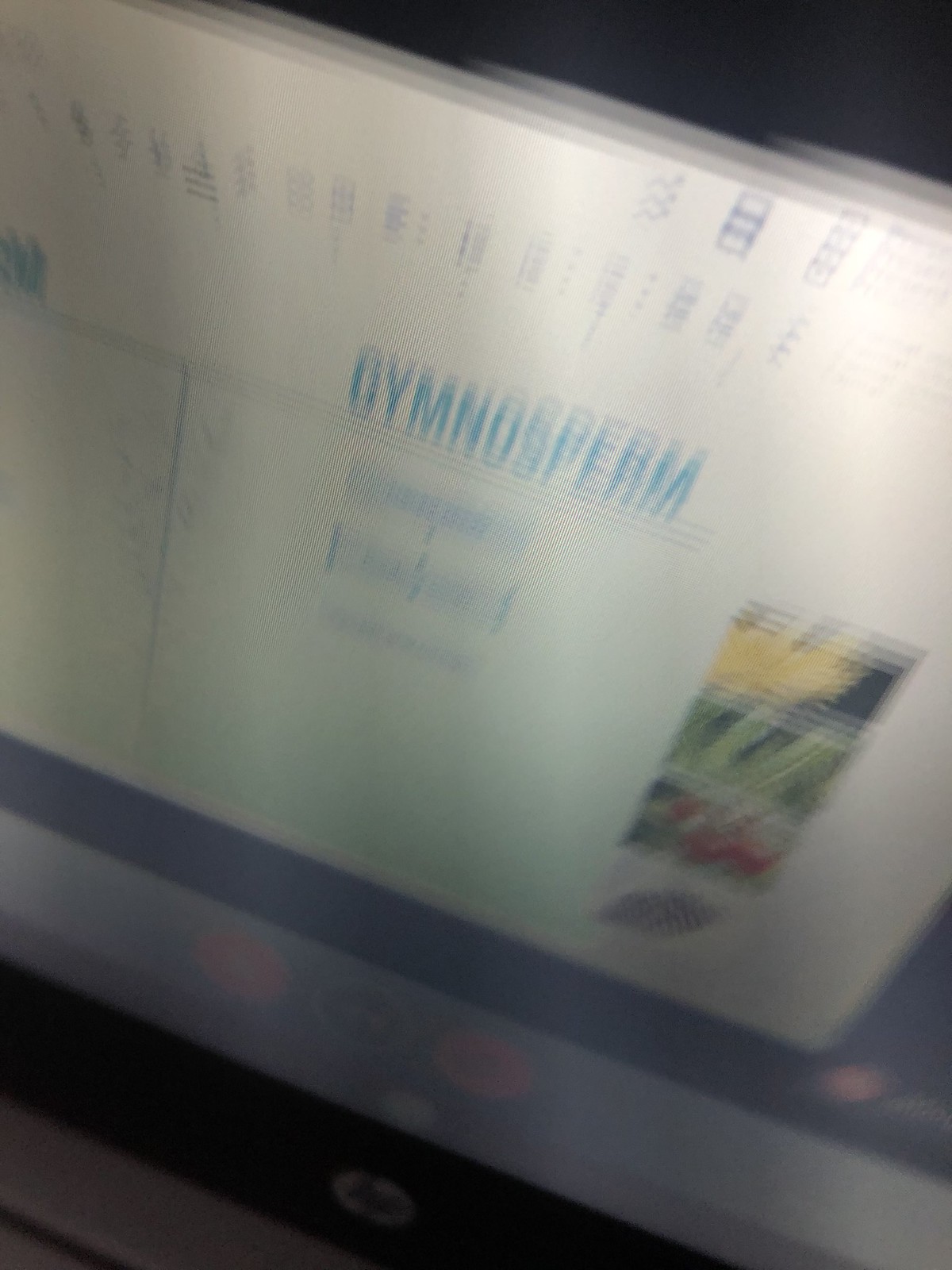The photograph captures a rectangular image predominantly featuring someone's computer monitor. The composition reveals that the left and right sides are longer than the top and bottom. Much of the image shows the computer screen displaying a web page, but the photograph is blurry and out of focus, as if the camera was in motion during the shot. The angle is slightly downward and frontal, exposing the top and a portion of the monitor, which is mostly out of frame. The center of the monitor displays a white web page with multiple pictures of flowers along the right side. The focal point of the page is large blue text reading "Jim, no sperm," accompanied by additional blue text that is too blurry to discern. The monitor's frame features a silver HP logo circle in the center.